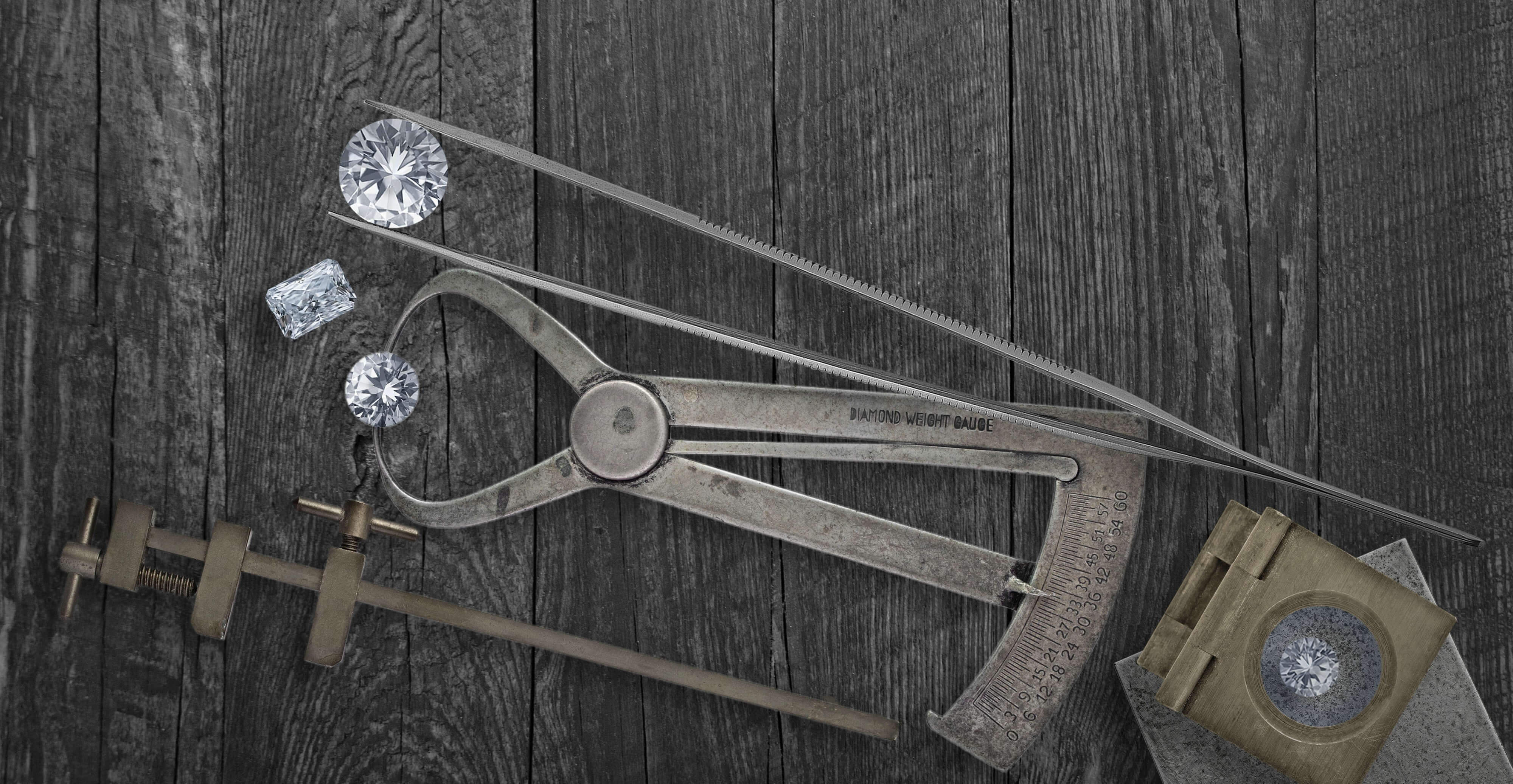The full-color photograph, professionally staged and horizontally rectangular, captures an intricately detailed scene set indoors on a dark, rich wooden table with visible cracks and spaces between the vertical planks. The main focus is a collection of vintage metal equipment, presumably used in the diamond trade, and several sparkling diamonds.

In the lower left corner, a complex apparatus extends towards the bottom middle. It features a long rod that begins at the left and curves towards the right, ending centrally. Attached to the rod are three rectangular pieces: two on the right and a smaller one at the end, which has a downward-pointing screw and an additional small piece extending from its top. The last rectangular piece also has a small copper component protruding from its top, extending left and right.

Central to the composition is another metal device, with thin clamps on the left holding a diamond. This device extends rightward, terminating in a protractor-like ruler. Just above this central device, another emerald-cut diamond is visible, positioned further left.

In the upper left corner of the image, three more diamonds of varying sizes are seen. One diamond, larger than the others, is securely held between two prongs of a long, metal-pronged device that crosses the protractor at its end and continues downward to the right. Below this, and almost touching the bottom right corner of the photograph, sits a square magnifying glass. Through it, another diamond is visible, resting on a gray material that extends off the image's lower right edge.

The juxtaposition of the polished, brilliant diamonds against the worn, older measuring instruments and clamps creates a striking contrast between new and shiny elements and vintage tools, emphasizing the meticulous and timeless nature of the diamond trade.